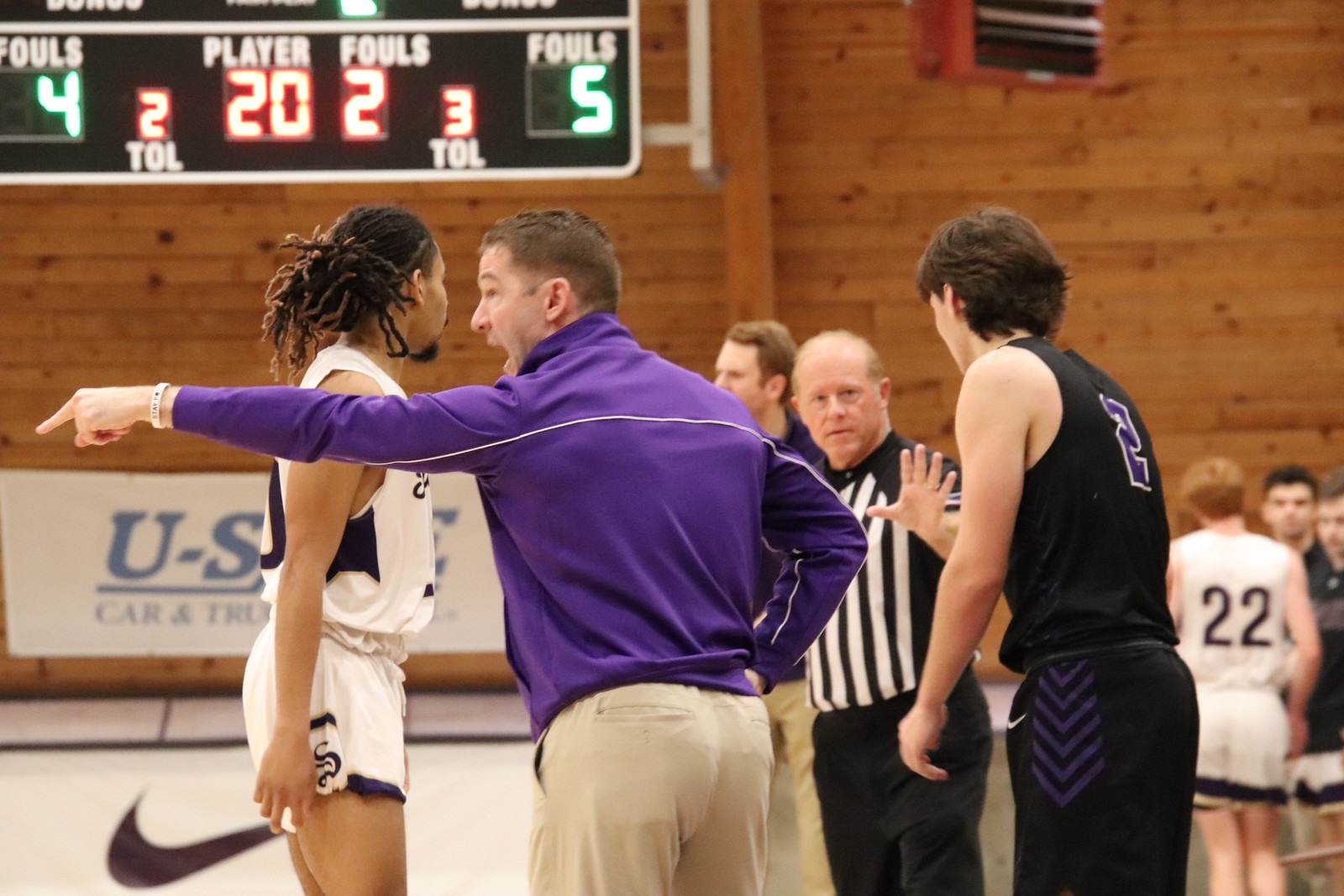In this image taken at a basketball game, the center of attention is an irate coach, dressed in a long-sleeved purple collared shirt and khaki pants. He is pointing aggressively towards the left, his mouth wide open as he shouts. To the coach's left stands an African American player in a white jersey and white shorts, wearing the number 22. The player, facing away from the camera, has braided hair pulled back into a ponytail. Near the coach's right side, there is a middle-aged referee, partially bald, extending his left hand with all five fingers visible, seemingly trying to calm the situation. The referee is mostly facing the camera. Further to the right is another player, wearing a black uniform with number 2 on it, and facing the referee. In the background, additional players are visible and the gym's wooden paneled wall can be seen. At the upper left corner of the image, a scoreboard displays various details like fouls and player numbers, indicating a heated moment in the game.